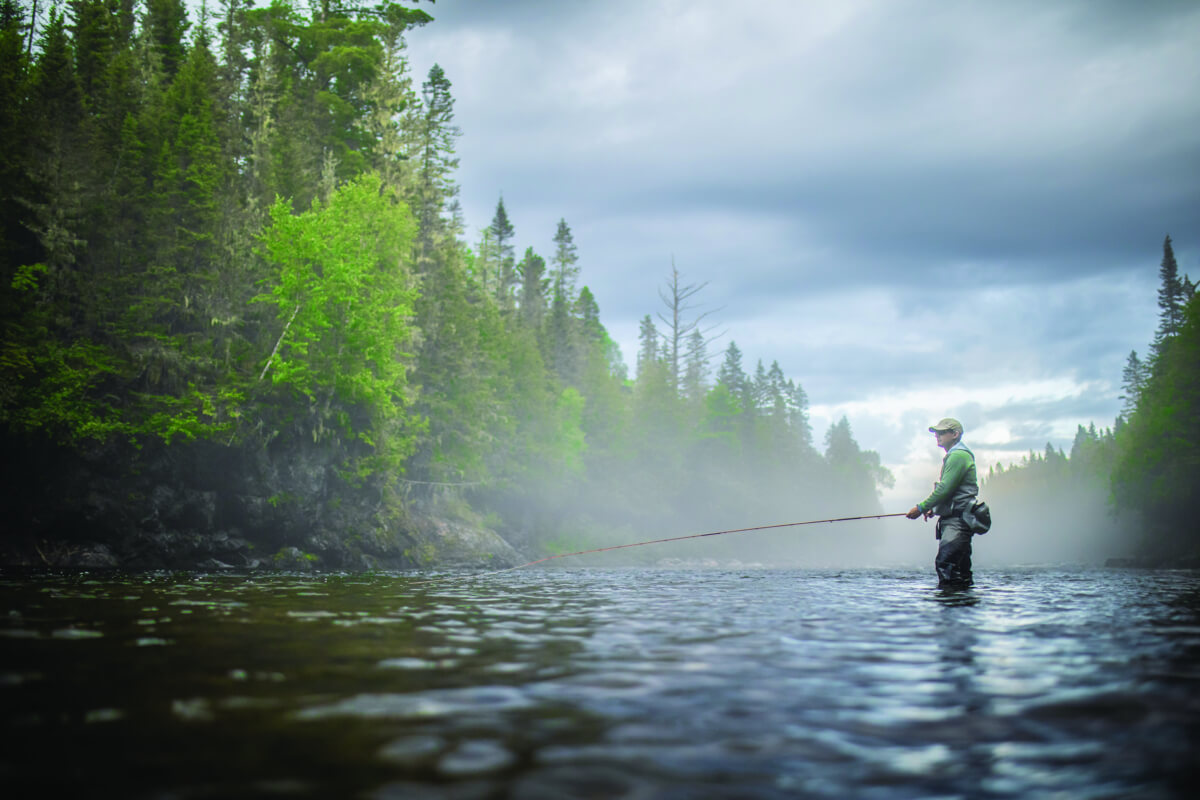In this photograph taken outdoors during the day, the sky is overcast with thick, dark grey clouds tinged with a blue hue, hinting at an impending rainstorm. The setting is a tranquil, shallow lake or river, with water coming just below the knees of a man who is fly-fishing. The man's long fishing pole cuts a striking figure against the moody sky. He is dressed in a green long-sleeved shirt and hip waders—rubber coveralls designed to keep him dry. He also sports dark-colored pants and a tan hat, with a utility pouch tied at his back near his waist.

The water appears mostly calm, with only slight ripples possibly caused by the man's movements and a gentle breeze. The shores are lined with dense trees, their colors varying from light lime to dark green. To the left, the trees are lighter in shade, while those on the right present a darker hue. The forest extends as far as the eye can see, creating a natural corridor flanking the water. In the distance, the scene becomes misty and hazy, perhaps due to humidity or fog, adding a mystical quality to the landscape. The left bank hints at a rocky terrain, which further encloses this serene fishing spot.